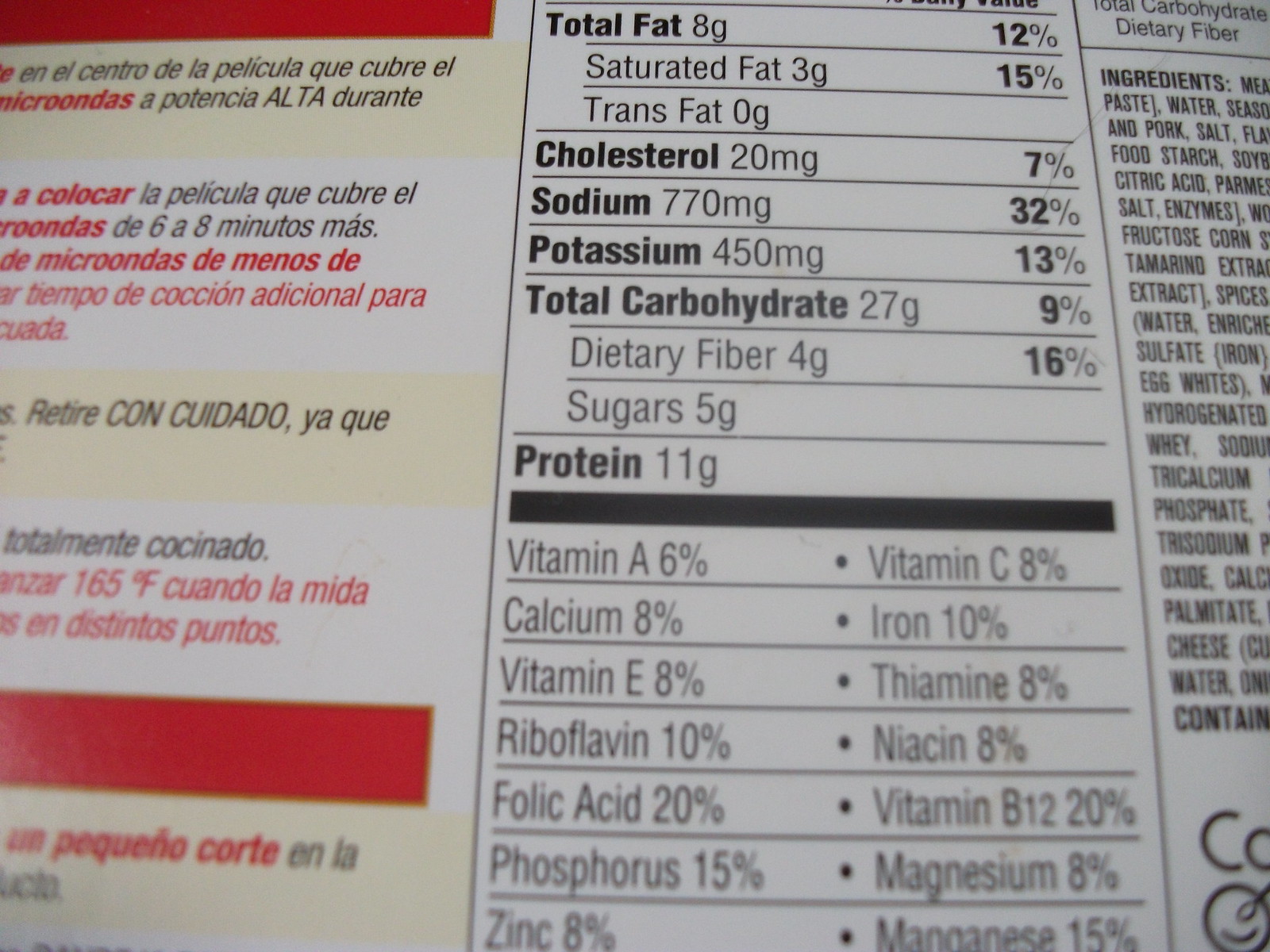This close-up image focuses on a food or drink packaging label. The left portion features a yellow and tan striped design with red banners and alternating red and black text in Spanish. In the top third of this section, a red border frames a white background with multiple lines of information. The lower part of the left section continues with lines of foreign text, some in red and black, all ending with another prominent red banner. The right portion of the label shifts to a more detailed nutritional breakdown on a white background. Black print highlights key nutritional information such as total fat, cholesterol, sodium, potassium, total carbohydrate, dietary fiber, sugars, protein, and several vitamins and minerals, including vitamins A, C, E, thiamine, riboflavin, myosin, folic acid, vitamin B12, phosphorus, magnesium, zinc, and possibly manganese, though the latter part is partially obscured. This section also includes a line separating the nutritional details from the ingredient list at the bottom, both continuing nearly to the bottom of the image.